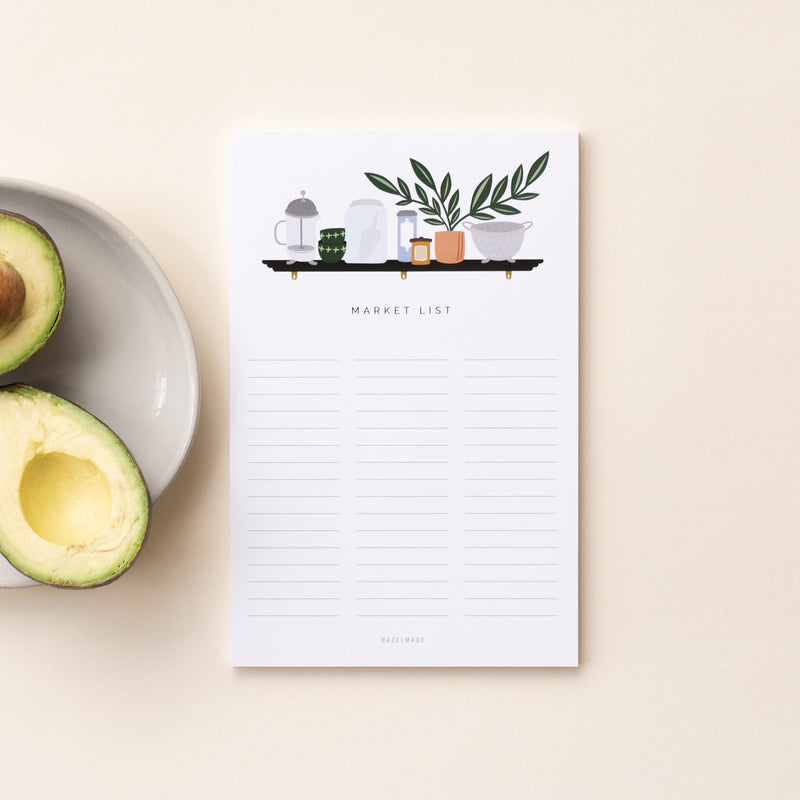The image depicts a vertically oriented notepad titled "Market List" in gray lettering at the top. The notepad is mounted on a white poster board, divided by gray lines meant for jotting down items. An artistic graphic adorns the bottom, featuring a shelf with various kitchen items: a blender, a pot with green leaves, multiple containers, and a jar with a spatula. Alongside the notepad is a ceramic white plate holding an avocado cut in half, displaying one half with the seed and the other half empty. This setup is placed on a white surface, illuminated by a light source. The phrase "hazel made" appears subtly at the bottom of the notepad.